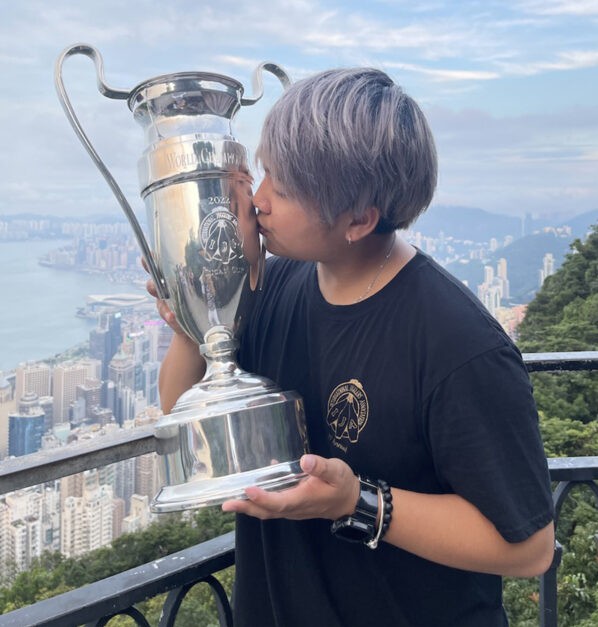In this detailed image, a person with short, silver-gray to light purple hair, possibly Japanese, is captured kissing a large silver trophy with "World Champion 2022" and bowling pins inscribed on it. Clad in a black t-shirt adorned with a golden emblem and a bowling pins graphic, they wear a smart watch, a black beaded bracelet on their left wrist, and an earring on their left ear. The person is standing on a high balcony, gripping the trophy with both hands, with his left hand beneath and his right hand supporting the back. The scene in the background reveals a sprawling urban landscape with numerous high-rise buildings, a river to the left, dark green trees, hills, and a blue sky scattered with clouds. The balcony itself has black metal railings, adding to the sense of elevation above the cityscape.